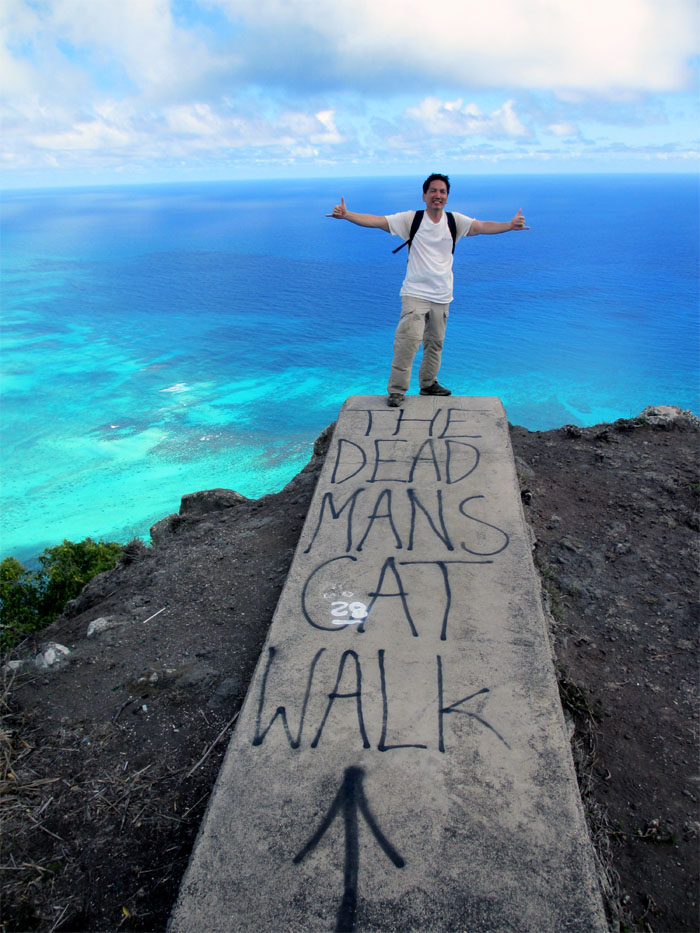This full-color outdoor photograph, taken on a mostly sunny day, captures the iconic Dead Man's Catwalk on the Kamahami Ridge Trail in Oahu, Hawaii. The vantage point, high above a breathtakingly beautiful blue ocean, reveals a striking coral reef in the background. Standing at the very edge of a concrete slab that juts out over the cliff, a man poses confidently. He is dressed in beige dockers and a white crewneck t-shirt, with the straps of a backpack visible on his shoulders. His arms are outstretched, hands forming the shaka gesture with thumbs and pinky fingers extended, embodying a relaxed, “all's cool” Hawaiian vibe. The slab beneath him is marked with the words "Dead Man's Catwalk" and an arrow pointing towards the precipice, seemingly written in felt-tip pen. The serene, green and blue ocean below stretches out to the horizon, meeting a partly cloudy sky, creating an awe-inspiring backdrop for this daring pose.